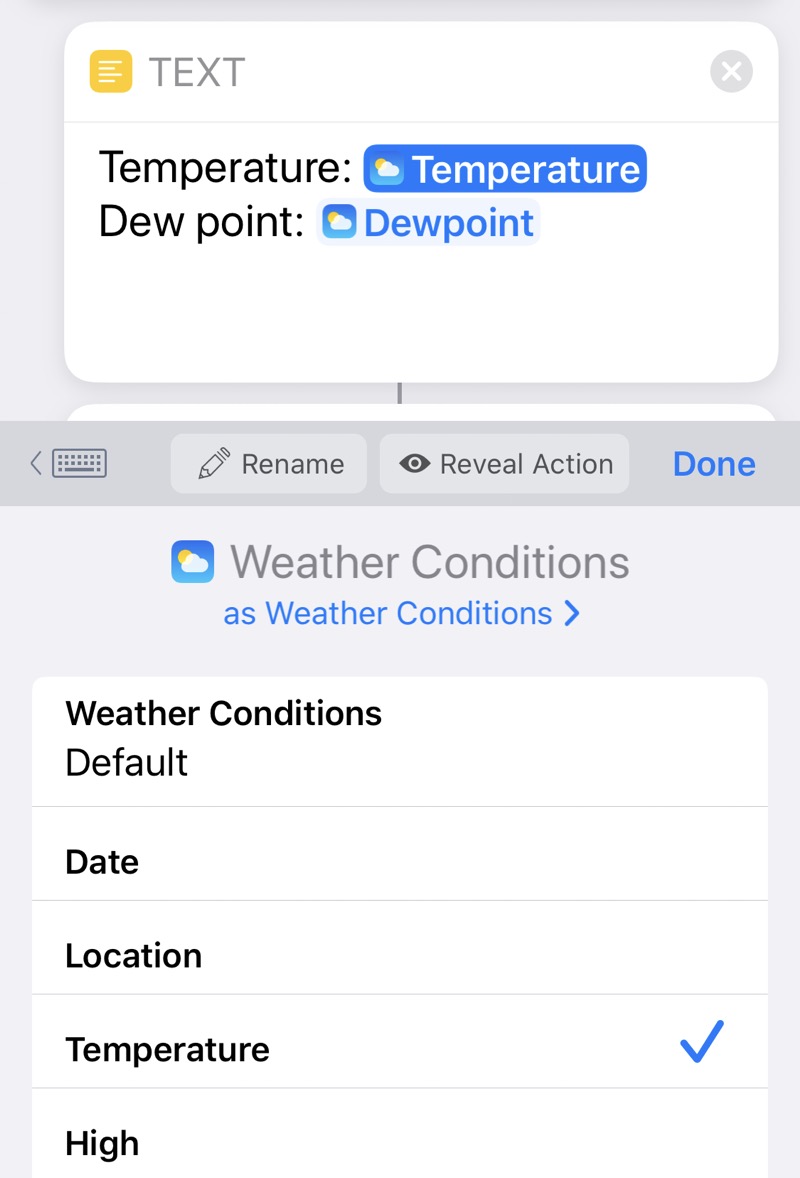This image captures the screen of a cell phone, prominently featuring a weather application interface. The screen is significantly taller than it is wide. At the very top, there is a white rectangle. Inside the top-left corner of this rectangle, there is a yellowish box containing five white horizontal lines stacked on top of each other, symbolizing a menu or list. Adjacent to this icon, the text "Text" is displayed.

In the top-right corner of the screen, a circular icon with an 'X' is visible, presumably to close or exit the current screen. Directly below this, the word “Temperature” is displayed, accompanied by a blue icon depicting a sun partially obscured by clouds, labeled "Temperature".

Further down, the term "Dew Point" is shown, next to the same blue sun-and-cloud icon, labeled "Dew Point". Below these, the background transitions to gray with a small arrow pointing to the left. This section includes icons for a keyboard, a pencil with the option labeled "Rename", and an eye icon with the text "Reveal Action". A blue button labeled "Done" is also present.

Beneath this section, the same image of a sun and clouds appears once more, with the text "Weather Conditions" beside a right-pointing arrow. This is followed by a white box containing various pieces of information: 

- The first line reads "Weather Conditions."
- The next item is "Default," followed by "Date," which is unspecified.
- The line "Location" is present but no specific location is provided.
- "Temperature" appears next, with a blue check mark to its right.
- Finally, the word "Hi" is displayed, without any accompanying text.

This concludes the content visible on the screen.